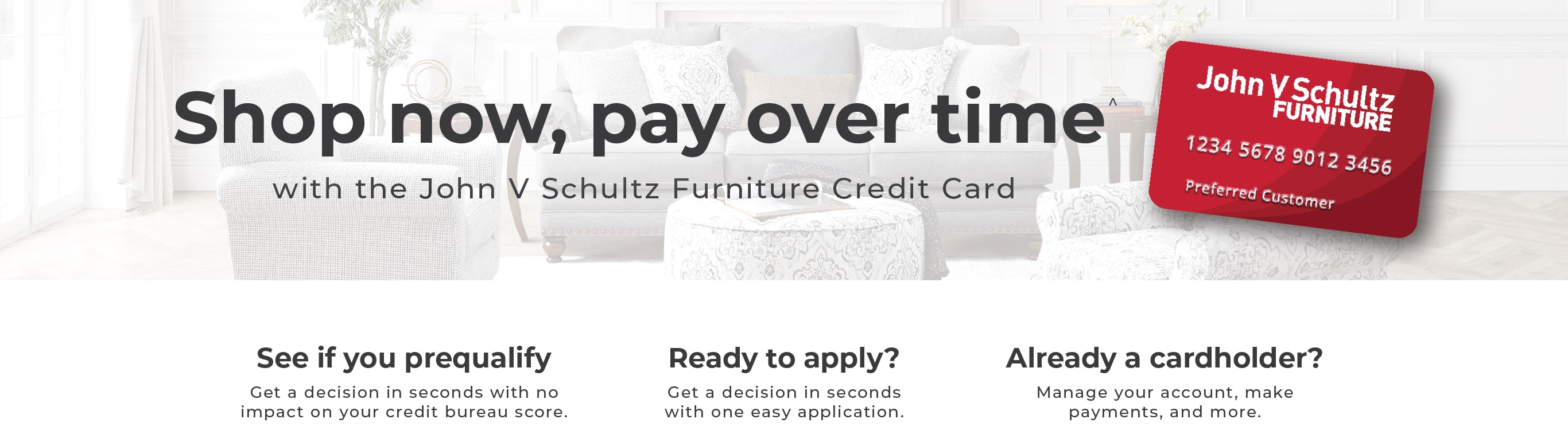The webpage features an inviting opportunity to apply for a furniture credit card. Dominating the top section is a banner set against a black and white photograph that exudes a cozy ambiance. The image showcases a stylish sofa adorned with throw pillows, accompanied by a round upholstered ottoman and a pair of occasional chairs. To the left, a window dressed in elegant treatments frames the scene, with a lush potted plant adding a touch of greenery to the minimalist decor.

Overlaying this serene backdrop is promotional text in bold black font that reads, "Shop Now, Pay Over Time with the John V. Schultz Furniture Credit Card." On the right side of the banner is a striking red credit card image, emblazoned with "John V. Schultz Furniture" in white font at the top. It features a sample 12-digit credit card number and lists the holder as "Preferred Customer."

Below the banner, the page is organized into three user-friendly tabs. The first tab, labeled "See if you Prequalify," encourages users to check their eligibility with the promise of "Get a decision in seconds with no impact on your credit bureau score." The central tab, "Ready to Apply," provides an easy access point for users to start their application, highlighted by the phrase, "Get a decision in seconds with one easy application." The third tab, "Already a Card Holder," serves existing customers with options to manage their account, make payments, and more.